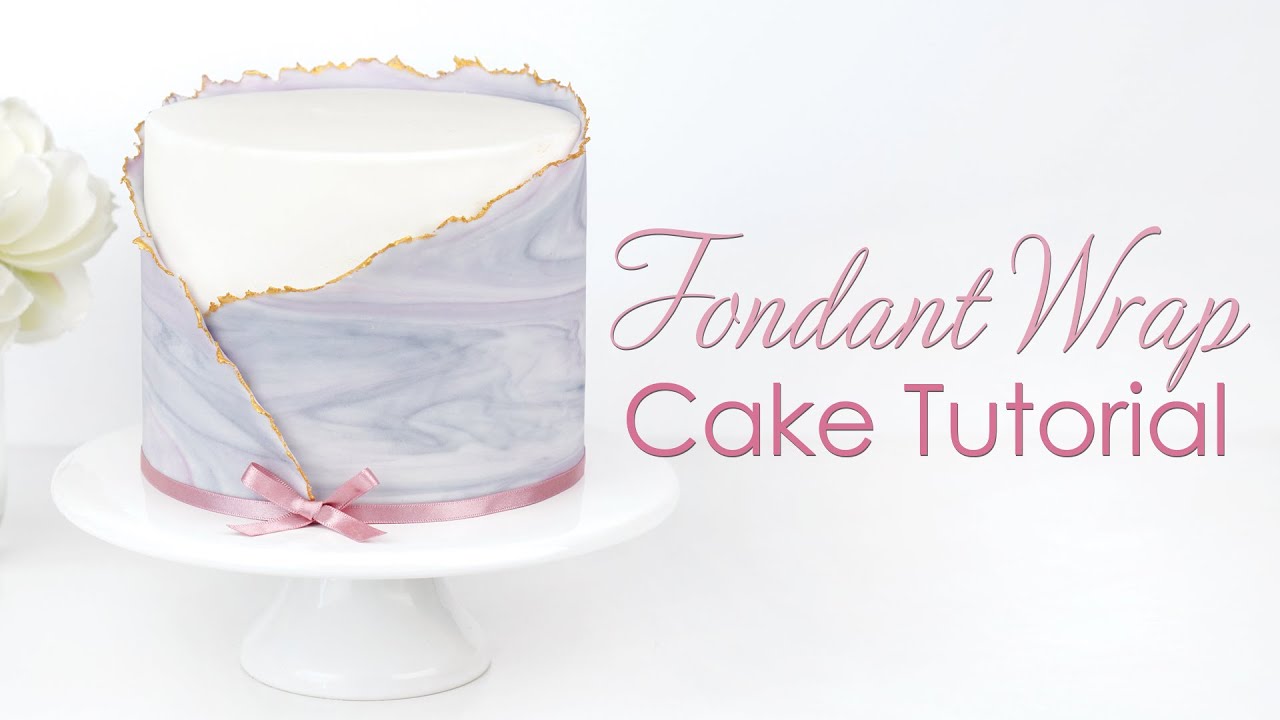This image features an advertisement for a "Fondant Wrap Cake Tutorial," prominently displayed in script font towards the right-center of the picture. The text, written in shades of pink—script font on top for "Fondant Wrap" and regular font beneath for "Cake Tutorial"—contrasts against a clean white background. To the left, there is a beautifully decorated cake placed on a white ceramic cake stand with a circular top and a triangular base. The cake itself is cylindrical and predominantly white, adorned with a striking fondant wrap featuring shades of blue, lilac, and baby pink, with splashes of gold at the edges. The fondant has a marbled texture that partially reveals the smooth white surface of the cake underneath. A pink ribbon encircles the base of the cake, adding a delicate touch, while a cut-off white flower is partially visible to the left of the cake, adding to the elegant presentation.